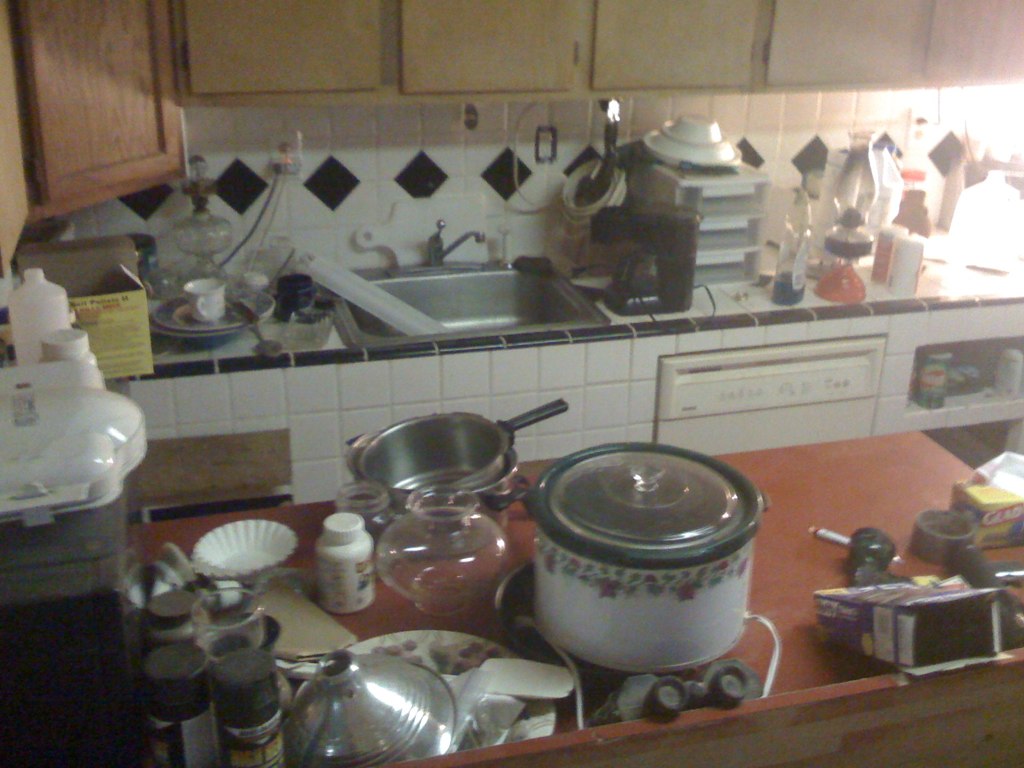The image portrays a highly cluttered kitchen with various items occupying the countertops, giving it a chaotic appearance. The upper cabinets are made of tan wood grain, adding a warm touch to the kitchen. A white tile backsplash with a distinctive black diamond pattern runs around the kitchen, adding a decorative element. A stainless steel sink is visible, partially filled with dirty dishes, and a mysterious white object sits inside the sink.

The countertop adjacent to the sink is crowded with numerous items, including dish soap, a coffee maker, and other miscellaneous kitchen gadgets. Below this area, a white dishwasher stands out, surrounded by more of the distinctive black diamond-patterned backsplash tiles instead of traditional lower cabinets.

On the opposite side of the kitchen, an orangey countertop houses a crock pot, a package of Glad trash bags, a box that appears to be empty, and coffee filters. The scene is further crowded with silver pans that have black handles, a waffle maker, and various other kitchen utensils creating an overall sense of disarray.